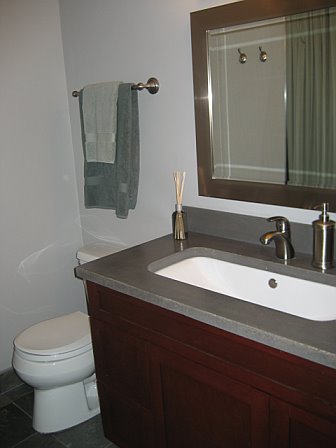The image captures a well-organized bathroom interior. At the bottom left corner, there is a standard white toilet. A towel rack adorned with a green towel and a smaller white towel is affixed to the middle of the top section of the wall. To the right, a sleek steel sink with a large rectangular white basin sits on a gray countertop. Adjacent to the sink, on the left side, is a decorative piece featuring sticks in a container. A matching steel hand soap dispenser is positioned to the right of the sink. 

The cabinetry beneath the sink is brown, complementing the overall color scheme. A mirror with brown outer edges hangs at the top right, reflecting part of the shower curtain. The walls surrounding the sink area are a soft gray, while the floor tiles carry a similar gray tone. The corner of the room, housing the toilet, is painted white, lending a crisp contrast to the gray elements. The towel rack is made of copper, adding a touch of warmth to the decor. The mirror reflects additional bathroom details, including the shower curtain.